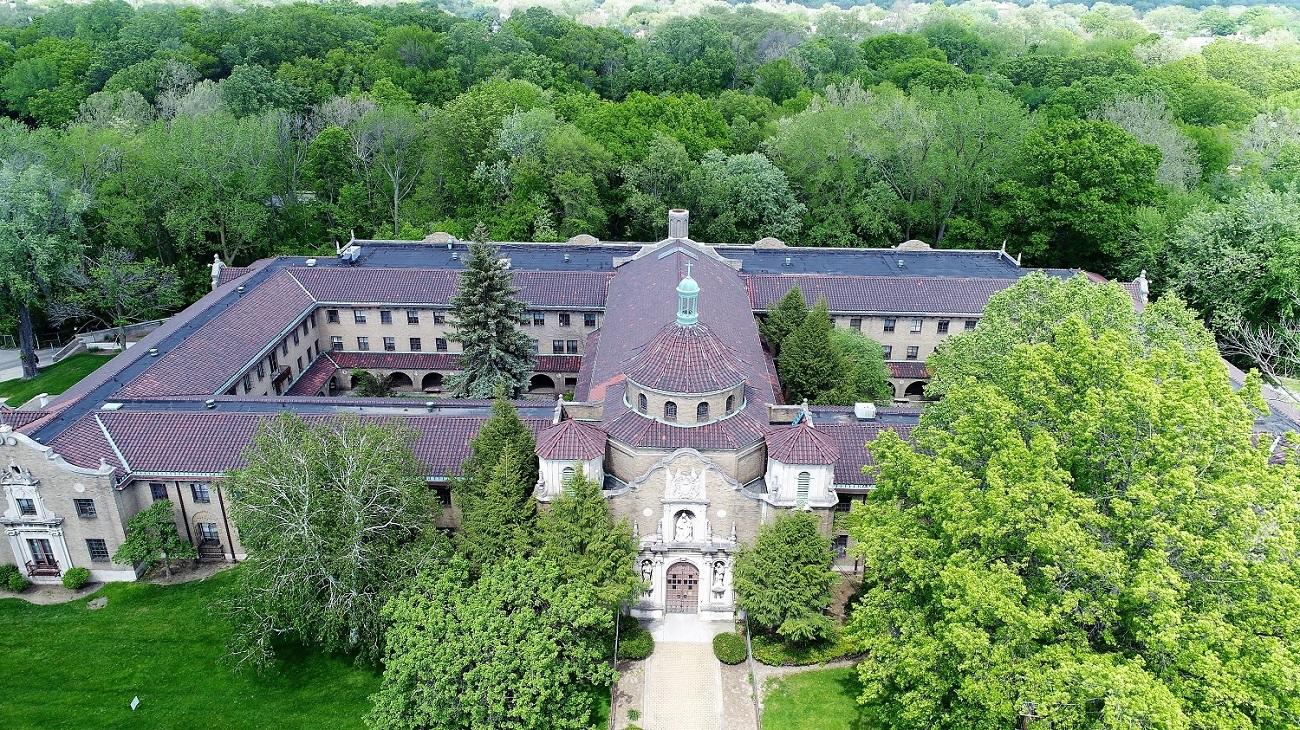This detailed aerial photograph captures a grand castle-like estate in a horizontal rectangular frame. Dominating the image is a massive building with a unique layout, resembling two connected squares or an elongated figure-eight. The structure's roof features a combination of colors, with a primary gray hue and accents of teal. The building's exterior is a light beige concrete, giving it a stately appearance, and it possibly functions as a hotel, church, or palace.

The estate encompasses a central courtyard, visible only in part, with lush treetops suggesting an inviting green space below. Surrounding the estate are vibrant green trees, creating a stark contrast and adding to the grandeur of the scene. The upper third of the photograph is filled with these trees, their bright green foliage contributing to the overall lushness of the landscape.

In the front of the building, a prominent tower, possibly reaching three stories, catches the eye with its gray roof. A wide, cream-colored sidewalk or driveway leads up to the main entrance at the ground level, flanked by orderly rows of trees and well-manicured grass. This path accentuates the geometric harmony and grandeur of the estate.

Overall, the image beautifully captures the blend of nature and architecture, showcasing the estate's sprawling design and picturesque ambiance.